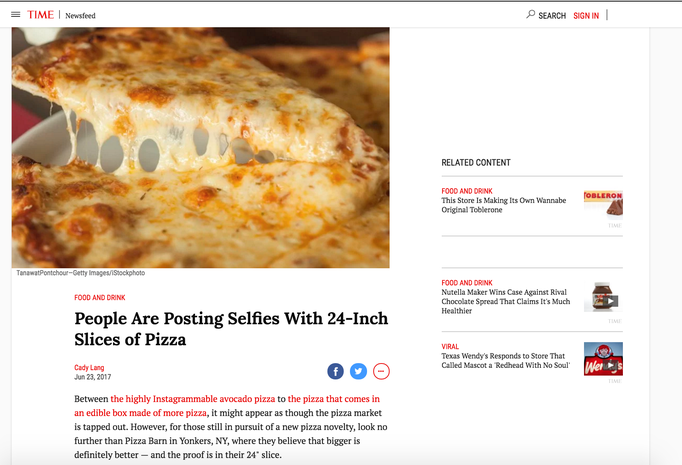A comprehensive visual guide to navigate the detailed website interface:

In the top-left corner, there's a compact icon of three horizontal black bars stacked vertically, typically representing a menu. Adjacent to this icon, the word "Time" is prominently displayed in red text. Directly next to this, a black vertical box labeled "Newsfeed" in black lettering. Across the top-right, there's a gray magnifying glass symbol, signifying the search function, followed by the word "Search" in black. Further to the right, a red "Sign In" button is visible.

Below this top navigation, on the left, there's a captivating close-up image of a cheese pizza. A slice is being lifted, with gooey melted cheese stretching impressively, tantalizing the viewer with its deliciousness. Beneath the pizza image, a caption reads "Getty Images stock photo." Directly below it, a red label states "Food and Drink," followed by a black headline, "People are posting selfies with 24-inch slices of pizza." 

Further down, in red, the byline reads "Katie Lang," and in black, the date "June 23rd, 2017." The article continues: 
"Between the highly Instagrammable avocado pizza to the pizza that comes in an edible box made of more pizza, it might appear as though the pizza market is tapped out. However, for those still in pursuit of a new pizza novelty, look no further than Pizza Barn in Yonkers, where they believe that bigger is definitely better—and the proof is in their 24-inch slice."

On the right side of the image, there's a section titled "Related Content" in black. Below this header, red subheadings "Food and Drink" introduce: 
- "The store is making its own wannabe original Toblerone."
- "Nutella maker wins case against rival chocolate spread that claims it's much healthier."

Additionally, under the "Viral" category: 
"Texas Wendy's responds to store that called mascot a redhead with no soul."